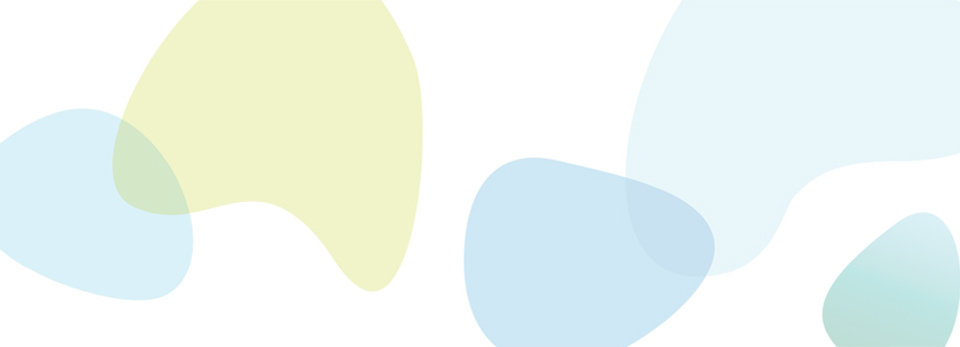On a plain rectangular white background, the image features multiple indefinite shapes in various colors: a pale blue, a deeper blue, a yellowish-brown, and two shades of green. The shapes are positioned primarily towards the four corners of the image and overlap in some areas. In the bottom right corner, a darker green shape intersects with a pale green one, creating a richer green at their intersection. Above this, a pale blue shape blends into the green. On the left side, near the bottom, there is another light blue shape that intersects with a yellowish-brown shape, creating a blend of colors. The blue shapes, described as resembling fingerprints, add depth and variation to the overall abstract design.